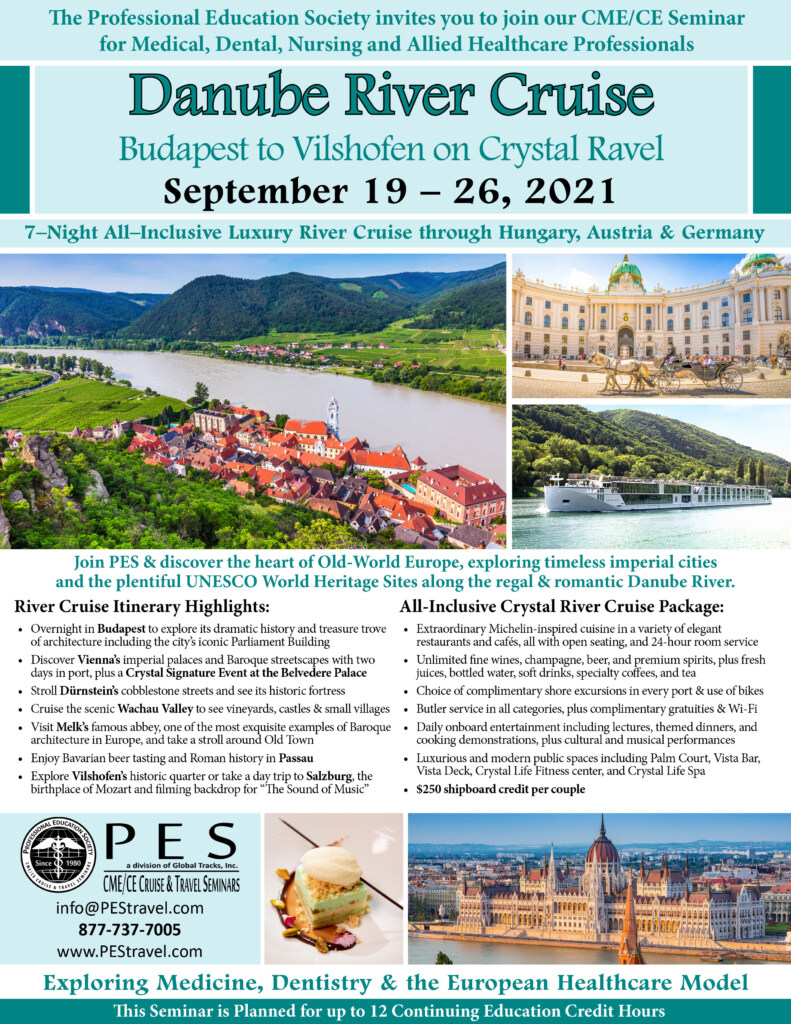This vertically oriented rectangular poster advertises a Danube River cruise from Budapest to Vilshofen, scheduled for September 19th through the 26th in 2021. The upper portion of the poster, set against a light green background, prominently features the text: "Budapest to Vilshofen on Crystal Ravel, September 19-26, 2021. 7-night all-inclusive luxury river cruise through Hungary, Austria, and Germany." It also mentions that the cruise is hosted by the Professional Education Society, inviting participants to join a CME/CE seminar for medical, dental, nursing, and allied health care professionals, offering up to 12 continuing education credit hours.

Below the header, the poster showcases several photographs, highlighting scenic views along the cruise route. One large photo captures the serene Danube River alongside a picturesque village where nearly every building sports a red roof. Two smaller images depict notable sites: one featuring a majestic white building with green domes, and another showcasing a two-story white riverboat adorned with expansive windows.

Further down, the poster features black print text detailing the cruise itinerary and amenities. At the bottom, three additional images display more of the landscapes and experiences awaiting passengers, including a close-up of a sumptuous dessert, illustrating the culinary delights to be enjoyed on board. The name of the sponsoring company is also included, underscoring the luxury and professional focus of the river cruise.